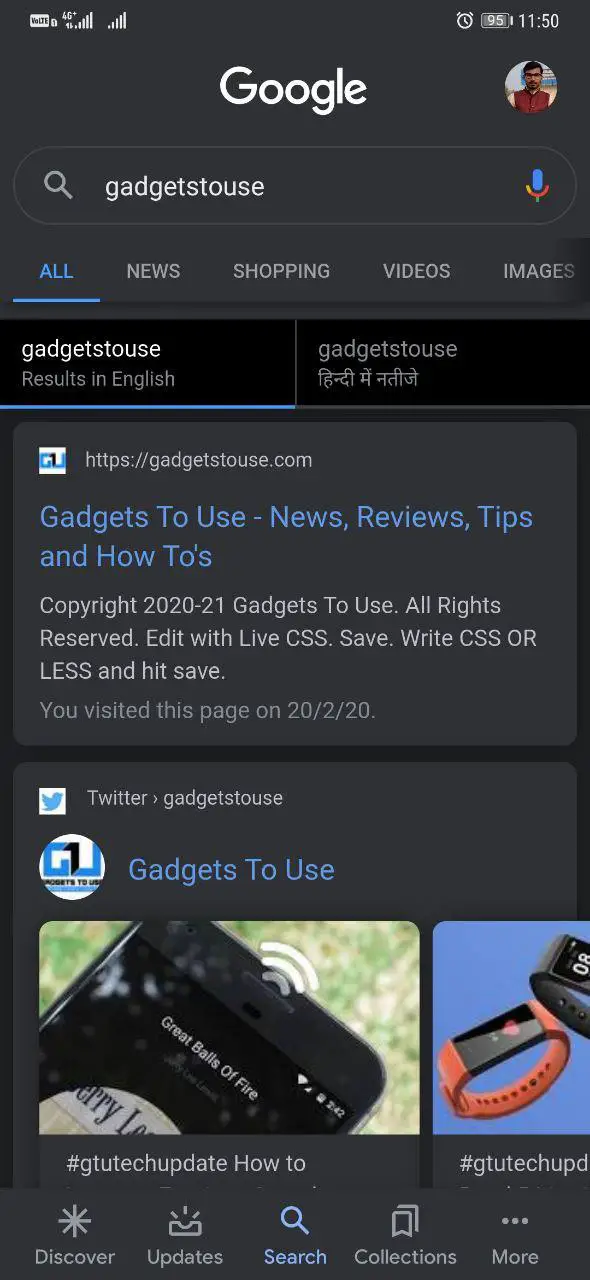This image captures a screenshot of a Google search result displayed on a phone, oriented in portrait mode. The screenshot, framed against a gray background, is about two to three times taller than it is wide. 

At the very top of the screen, several icons are visible. The first icon is unidentifiable, followed by a series of network status icons, all indicating a full signal. Further to the right are an alarm clock icon, a horizontal battery icon showing a 95% charge with an internal gray meter and white numbers, and a clock displaying the time as 11:50.

Directly beneath these icons, a white header features the word "Google" alongside an avatar of a person with black hair wearing a red vest. Below this header is an elongated, oval-shaped search box containing the search query "Gadget Status." Under the search box, several category options are listed including "All," "News," "Shopping," "Videos," and "Images"—all in white font except for "All," which is highlighted in blue with a blue underline.

Following this search tool, a black box appears with the text "Gadget Status results in English," accompanied by its translation and a foreign symbol. Below this, a horizontal gray rectangle displays the link for "Gadget Status" in white text, followed by a header in blue and a description in white.

Continuing down, there is a Twitter search result titled "Gadgets to Use," featuring two thumbnail images of different gadgets.